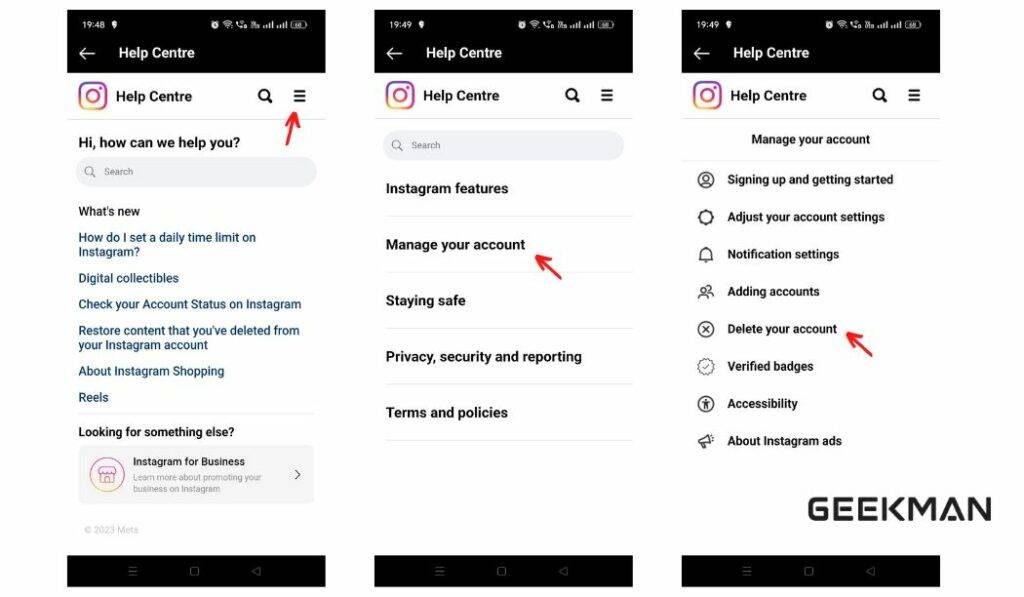**Detailed Instructional Guide for Deleting Your Instagram Account by Geekman**

This side-by-side instructional image provides a step-by-step guide on how to delete your Instagram account, created by Geekman, whose watermark appears in large block capital letters in the lower right-hand corner of the complete image.

1. **First Step - Accessing the Help Center:**
   - The first image displays the Instagram Help Center with the query prompt, "Hi, how can we help you?".
   - An arrow points to the 'hamburger' menu (three horizontal lines) located in the top-right corner. 
   - Options under this menu include sections like "What's new?", "How do I set a daily time limit on Instagram?", "Digital protocols", "Check your account status", among various other suggestions for assistance.

2. **Second Step - Navigating to 'Manage Your Account':**
   - Upon clicking the hamburger menu, the second image reveals an expanded list of options.
   - The categories available are "Instagram Features", "Manage Your Account", "Staying Safe", "Privacy, Security, and Reporting", and "Terms and Policies". 
   - A red arrow in this image highlights the "Manage Your Account" option.

3. **Third Step - Selecting 'Delete Your Account':**
   - Selecting "Manage Your Account" leads to a new set of options, as illustrated in the third image.
   - These options include "Signing Up and Getting Started", "Adjust Your Account Settings", "Notification Settings", "Adding Accounts", "Delete Your Account", "Verified Badges", "Accessibility", and "About Instagram Ads".
   - A red arrow specifically indicates the "Delete Your Account" option.

This detailed image guide helps users understand each step required to delete their Instagram account, with clear visual cues and instructions.